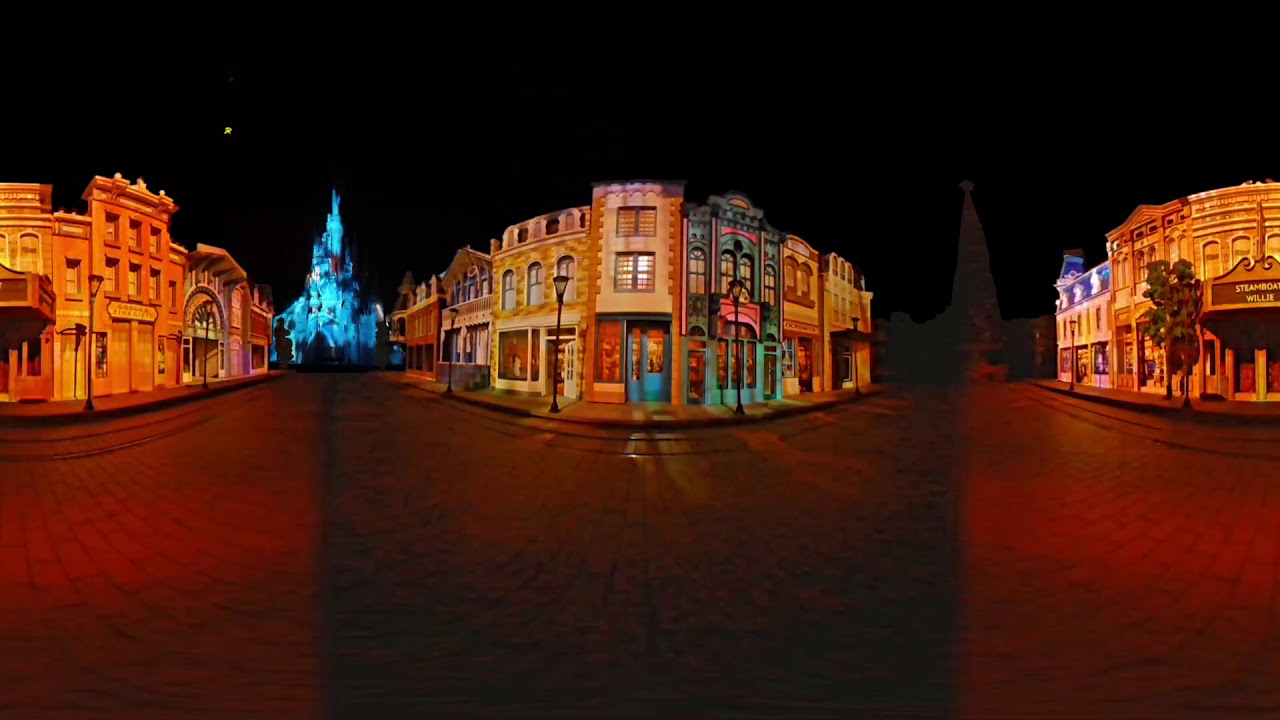This nighttime photograph, styled with a wide-angle lens that curves the scenery, captures a deserted Disney World scene. Centered in the background is the iconic Magic Kingdom castle, bathed in ethereal blue lights, which enhance its grandeur. The foreground presents a wide, deep red cobblestone walkway, almost courtyard-like, bordered by lampposts resembling gas lamps and dotted with a few sparse trees. 

Spanning from the left to the right of the image, multiple buildings, styled to resemble an old wild west town, stretch across. To the left, a three-story building with a prominent arch features orange highlights and a distinctive sign. In the middle stands another three-story white building with brick accents, distinguished by a blue door at its corner and green doors along its side. 

Next to it, a building houses the Steamboat Willie Theater, proudly displaying its name above, and is fronted by a small tree. Further to the right, another two-story building sits adjacent to a second two-story structure with a store at its bottom. All these buildings are illuminated in rainbow, neon hues—blue, purple, and red—adding a magical vibrance to the scene. 

The street is empty, with no people, enhancing the surreal quality of this Disney World image. The black sky above is mostly void except for a single, twinkling star in the upper left corner, adding a touch of celestial charm. This whimsical, seemingly otherworldly image encapsulates the enchantment of Disney World under a starry night.